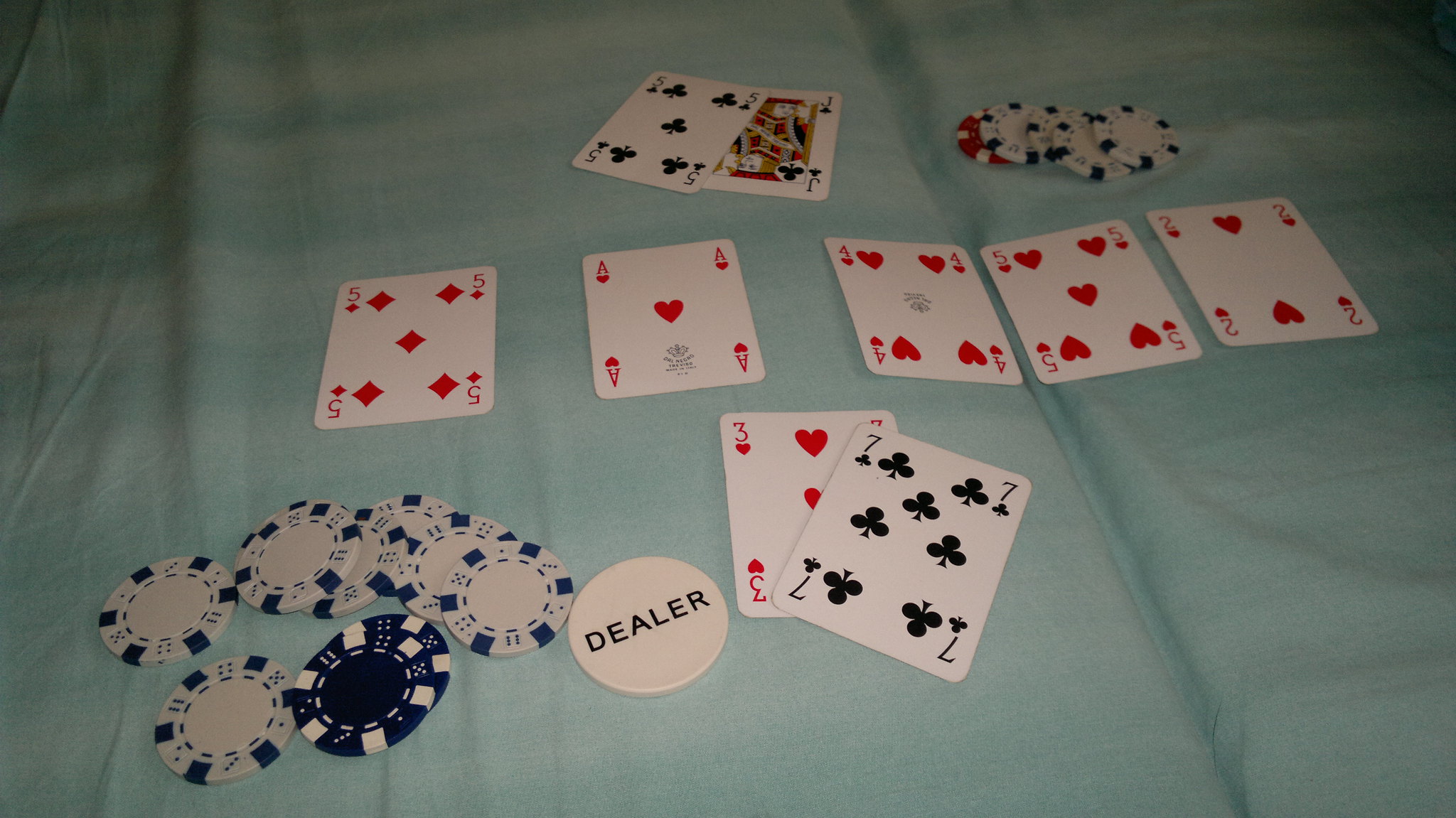This photograph showcases an intimate scene of a card game taking place on a table covered with a blue cloth, situated within a home. The table is arranged for a game of Seven Card Stud, indicated by the five community cards laid out: the Five of Diamonds, Ace of Hearts, Four of Hearts, Five of Hearts, and Two of Hearts.

In the foreground, a black chip labeled "Dealer" is prominently placed next to the cards closest to the viewers, signaling the dealer's position. The dealer has two cards in front of him: the Three of Hearts and Seven of Clubs. His opponent also displays two cards: the Five of Clubs and Jack of Clubs.

Chips are scattered around the players, suggesting the ongoing nature of the game. The dealer has a modest but significant collection of chips, while the opponent's stack is visibly smaller, consisting of three white chips and one red chip.

Analyzing the cards reveals that the dealer is poised for a victory. Combining the dealer's cards with the community cards could form a flush or even a straight flush, assuming the rules permit Aces to be both low and high. In this case, the dealer would hold a powerful hand: Ace, Two, Three, Four, Five of Hearts.